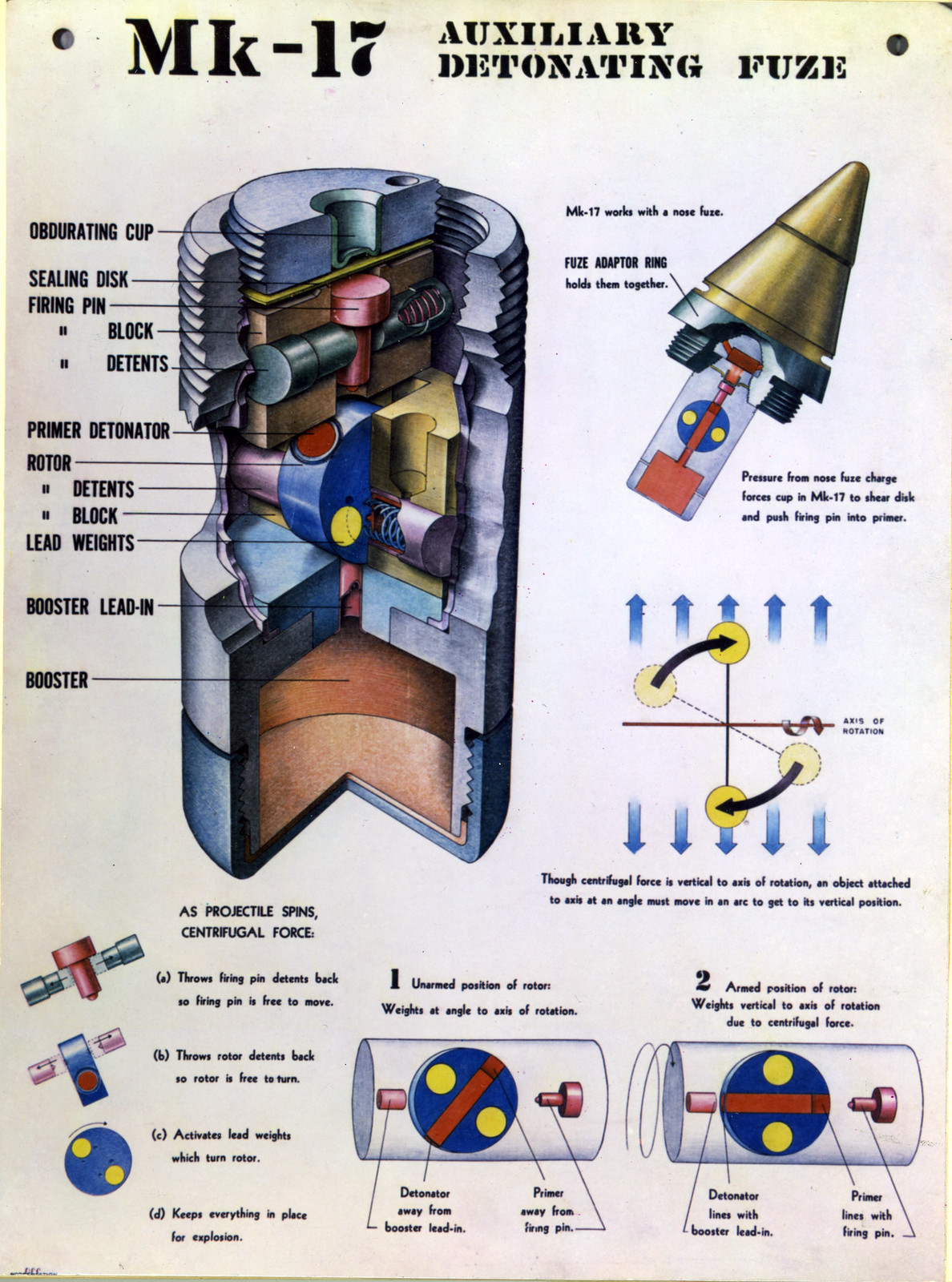The image is a tall, rectangular schematic diagram of the MK-17 Auxiliary Detonating Fuse, displayed on off-white paper that fades to a more beige, yellowy color at the edges. There are two holes punched into the paper's top left and right corners. Between the holes, in bold black lettering, it reads "MK-17 Auxiliary Detonating Fuse." Below this text, on the left side, there is a large, colored cross-sectional diagram of the fuse showing its internal components. The fuse's silver chamber reveals intricate parts such as the obturating cap, sealing disc, firing pin, block, dents, primer detonator, rotor dents block, lead weights, booster, and lead-in booster, all meticulously labeled.

To the right of the cross-section, a gold, cone-shaped piece of the fuse is illustrated, representing the cap. Additionally, the bottom right corner features a diagram depicting centrifugal force during projectile spin. This diagram includes a round tube with blue circles divided by yellow dots and intersected by red lines. Several smaller diagrams with explanations written in black font are present below the main images and to the right, providing detailed insights into various operational aspects of the fuse. One specific diagram outlines directions with arrows indicating left, right, up, and down movements, crossed by an 'X' in the middle, further enhancing the technical illustration.